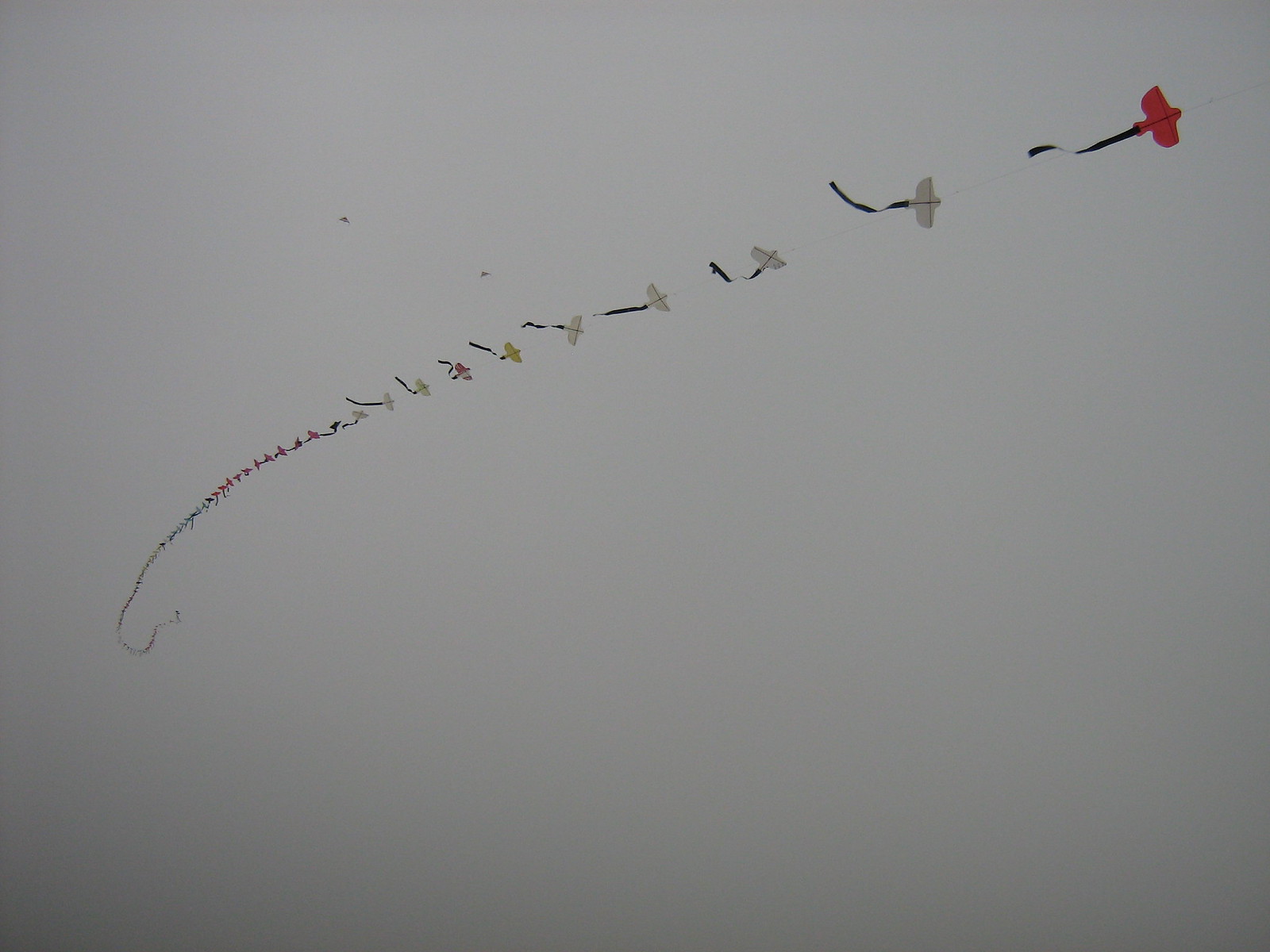This digital photograph captures a striking scene of a string of bird-shaped kites soaring into a vast, grey sky devoid of any blue or texture, resembling one continuous cloud. The kites form a long, diagonal line starting from the upper right corner and descending towards the lower left. The most prominent kite, at the starting point, is a vibrant red bird with a trailing black streamer. As the kites progressively get smaller and higher in the sky, they follow a color sequence of red, white, white, white, white, white, yellow, red, white, white, white, black, red, before becoming indistinguishable due to distance. The nearly invisible string connects each kite, blending seamlessly into the overcast backdrop, making it appear that the kites are freely floating in the sky. Some stray shadows, perhaps from birds or additional kites, add subtle depth to this monochromatic yet captivating skyscape.